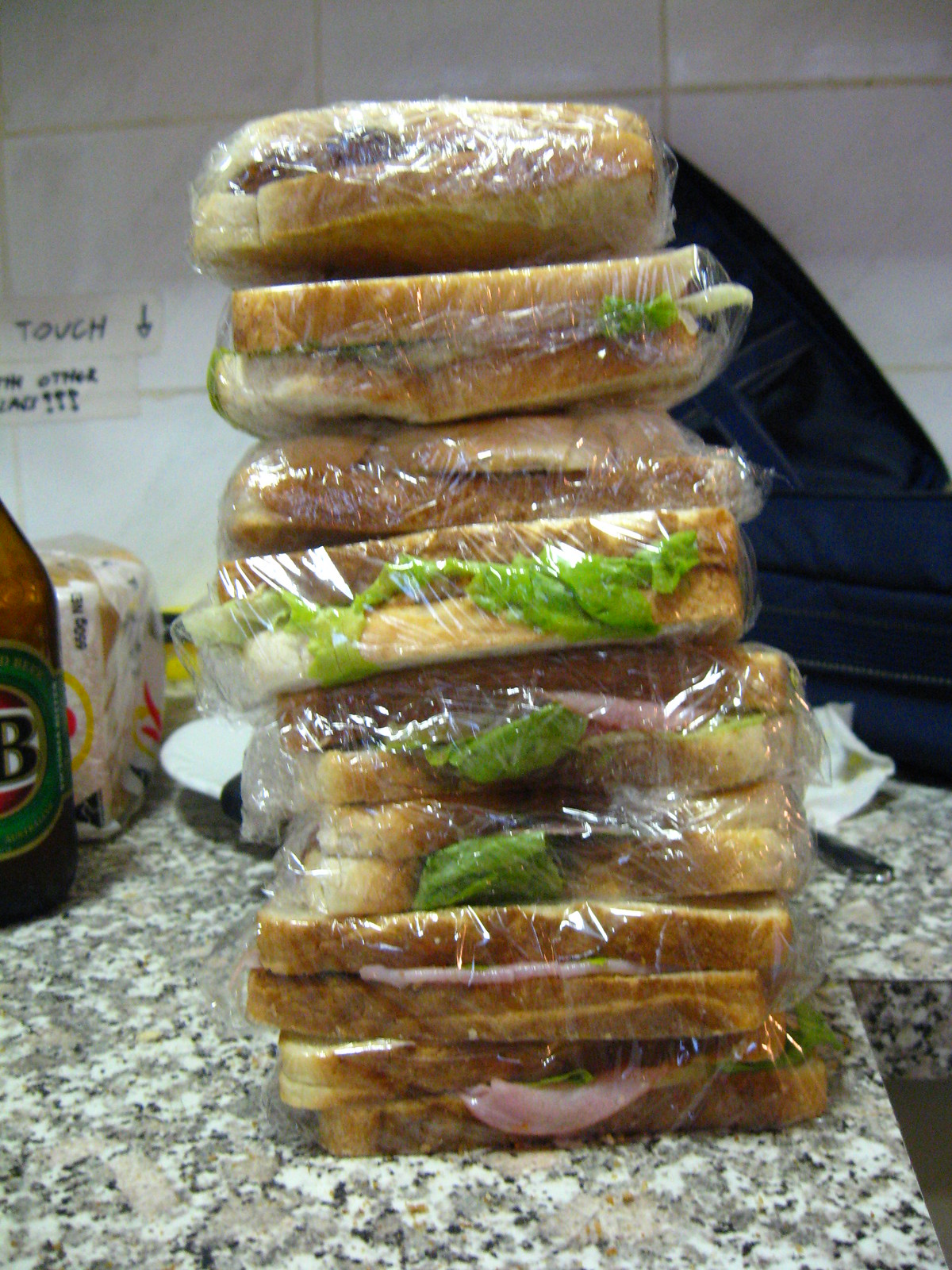This color photograph depicts a kitchen scene centered around a sturdy, granite-grey countertop. Piled neatly on the surface are around eight sandwiches, each made up of two slices of white bread and filled with visible lettuce and processed meat, likely ham. Each sandwich is individually shrink-wrapped in cling film to keep them fresh. To the right of the stack of sandwiches sits the partial view of a beer bottle, identifiable by its green label with a prominent "B" in the middle. Additionally, a loaf of bread and the handle of a knife are visible on the countertop. In the background, a white tiled wall features a handwritten sign with partial legible words including "touch" and "other," accompanied by an arrow pointing downwards. A cup adorned with multi-colored flowers is also visible, adding to the kitchen's details.